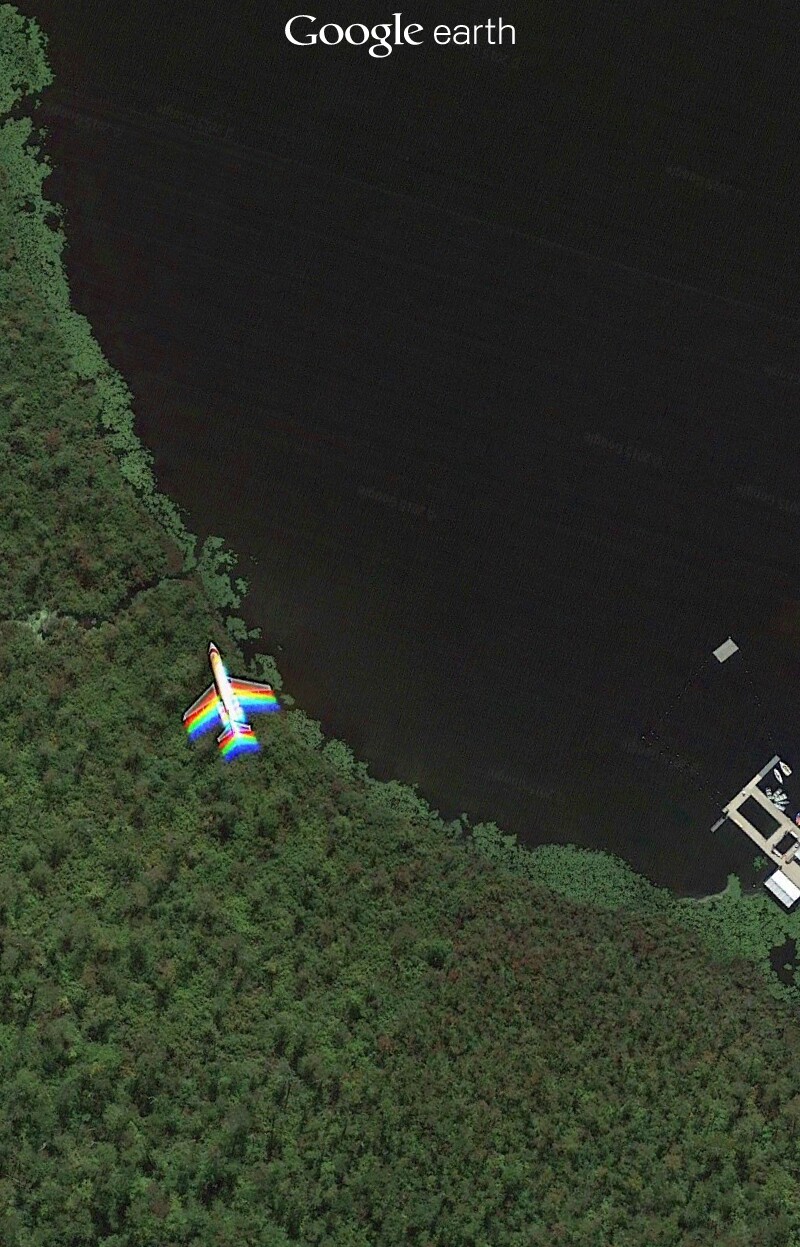This is a vertically rectangular frame featuring an aerial view dominated by a dark black lake, bordered by lush greenery. The top of the image is labeled "Google Earth" in two distinct fonts, with "Google" in a capitalized G and "Earth" in lowercase letters. A dock extends into the water from the lower right edge, where several small boats are moored. The dense, wooded area surrounding the lake is a vibrant mix of green hues with occasional splashes of red. An airplane, with red, orange, white, and blue stripes on its wings and tail, flies towards the upper left corner, leaving behind rainbow highlights.